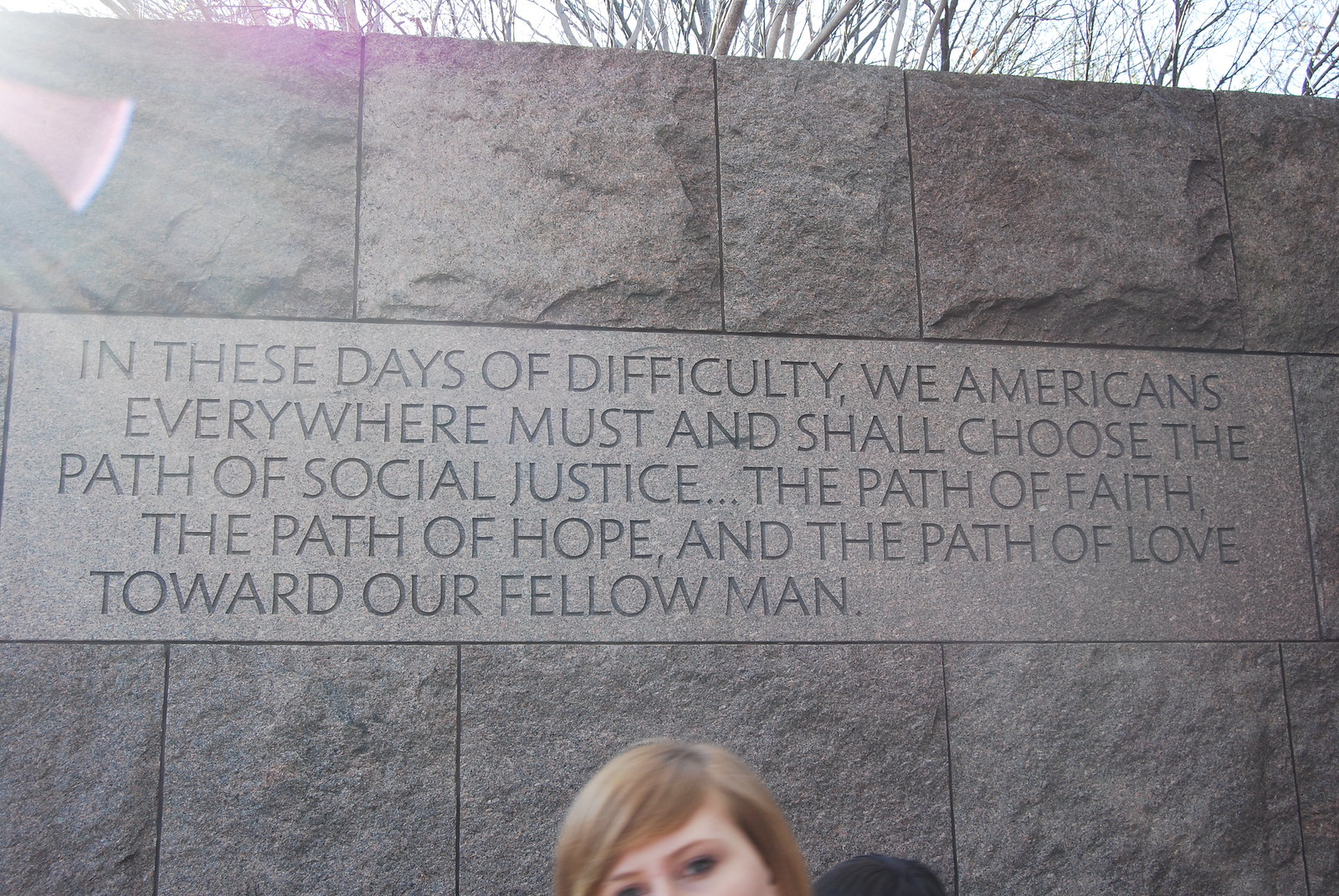In the image, a woman with short, blonde-brown hair and blue eyes stands in front of a gray stone wall. The wall features textured tiles and blocks, with a smoother, lighter gray rectangular section in the center. Carved into this smooth section are the words: "In these days of difficulty, we Americans everywhere must and shall choose the path of social justice, the path of faith, the path of hope, and the path of love toward our fellow man." The top of the woman's head, part of her face up to her cheek, and a glimpse of her dark blue shirt are visible in the foreground. Above the wall, there is a faint purple light and a background of white sky with thin, brown, leafless tree branches peeking through.